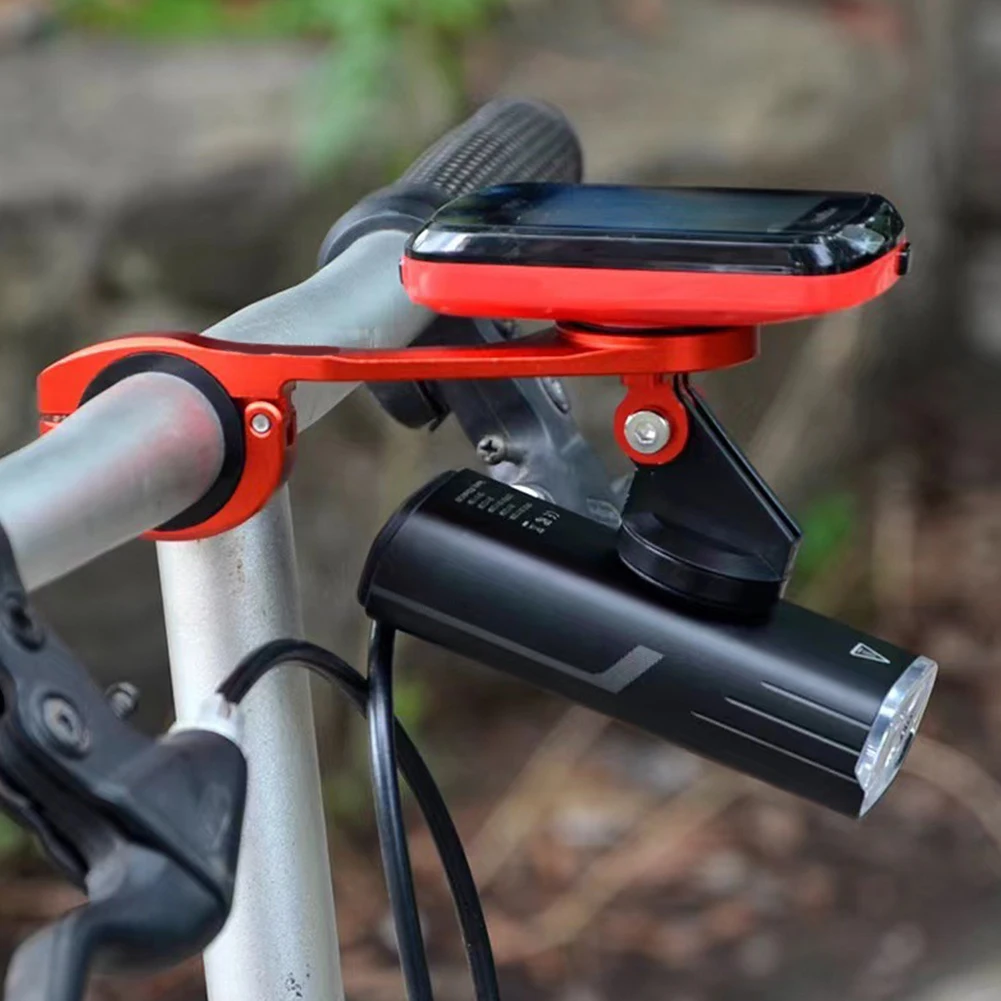A close-up photograph captures the intricate details of a scooter's handlebars. The handlebars are predominantly silver with black grips. On the right side, a black brake lever with an attached wire is visible in the bottom left corner of the frame. Adjacent to it, another wire leads to a compact device affixed to the handlebars using a red clip. This device features a small screen encased in a red and black housing. Below the screen, a sleek black light is connected via a silver screw. The background of the image is an out-of-focus natural setting, providing a contrasting backdrop to the detailed machinery in the foreground.